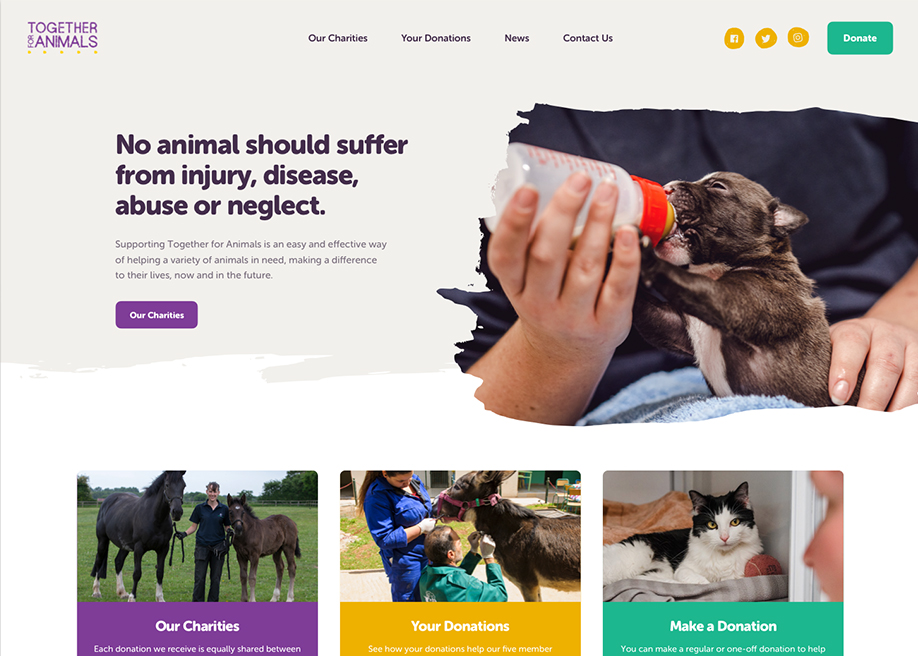This is a screenshot of a website that features a two-toned background: light gray on the top half and white on the bottom half. In the upper left corner, there is a dark blue logo for the website that reads "Together for Animals," accompanied by dark blue dots underneath. At the center top, the navigation menu in black font provides clickable options labeled "Charities," "Your Donations," "News," and "Contact Us." To the right of these options, there are three yellow circular social media icons: one for Twitter, another for Facebook, and an unidentified third icon. Adjacent to these social media icons, a gray button with "Donate" written in white stands out.

On the light gray upper section of the page, a bold black font headline on the left reads, "No animal should suffer from injury, disease, abuse, or neglect." Beneath this headline, regular black font text elaborates, "Supporting Together for Animals is an easy and effective way of helping a variety of animals in need, making a difference to their lives now and in the future." Below this text, there is a purple button labeled "Our Charities" in white.

To the right of this text block, an endearing photograph captures Caucasian hands holding a baby bottle and feeding a small, adorable gray puppy with a white chest. The puppy is seated on a towel on the person's lap, adding to the heartwarming nature of the scene.